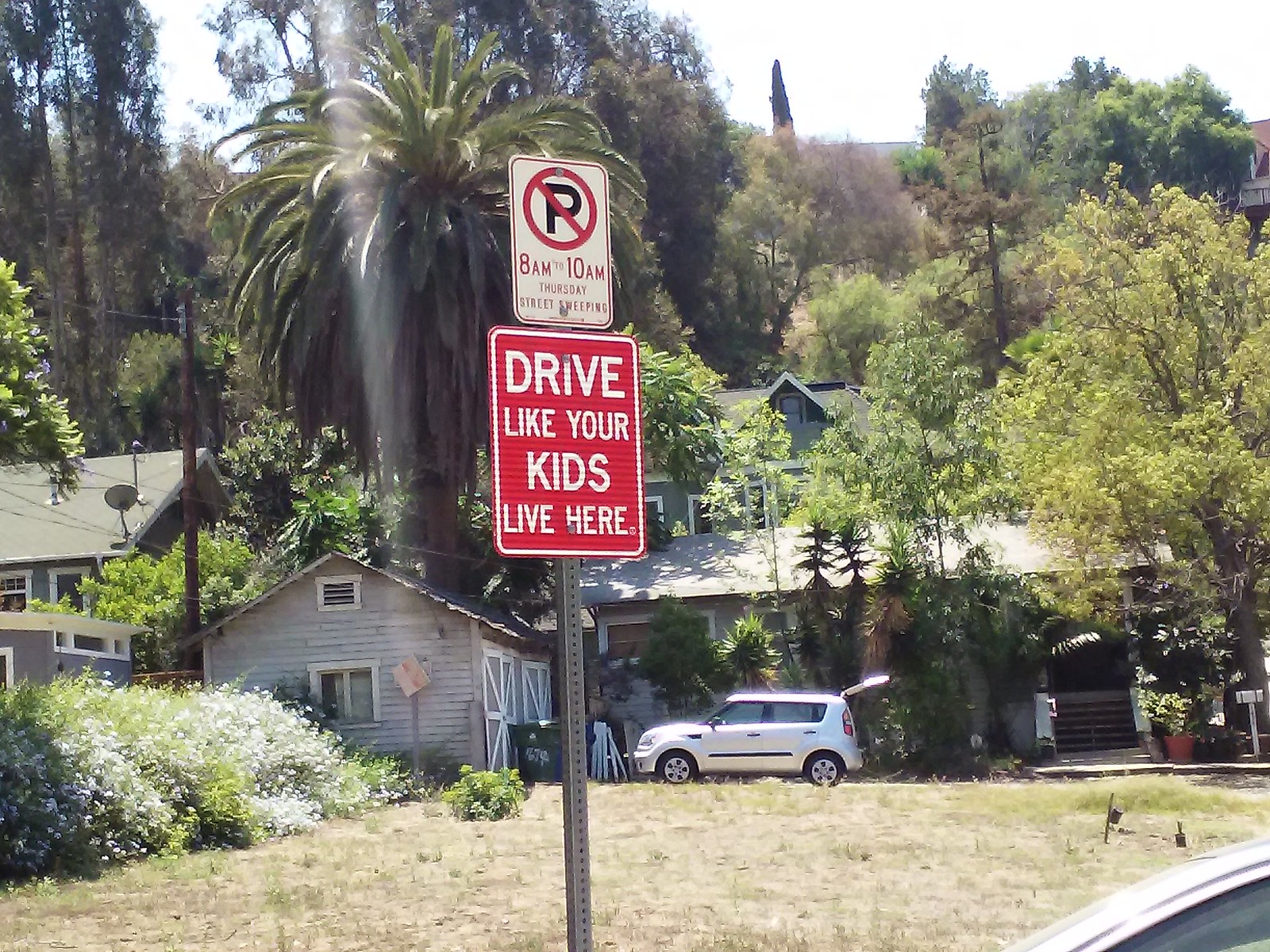The image captures a sun-drenched neighborhood scene, likely in a tropical or semi-tropical location such as Florida, California, or even Hawaii, indicated by the presence of lush palm trees. Dominating the foreground, a silver pole supports two signs: the upper one is a vertical white rectangle featuring a black 'P' crossed out diagonally, with red text specifying "8 a.m. to 10 a.m. Thursday Street Sweeping," while the lower, larger red rectangular sign reads "Drive Like Your Kids Live Here" in bold white letters. The terrain surrounding the sign showcases a yard with predominantly dry, brownish-green grass, hinting at hot weather conditions. An SUV, possibly a white Kia Soul with its hood open, is parked near a gray house with a garage, set against a backdrop of dense greenery including shrubbery and additional trees. A noticeable sun glare at the top of the image imbues the scene with a bright, radiant quality.